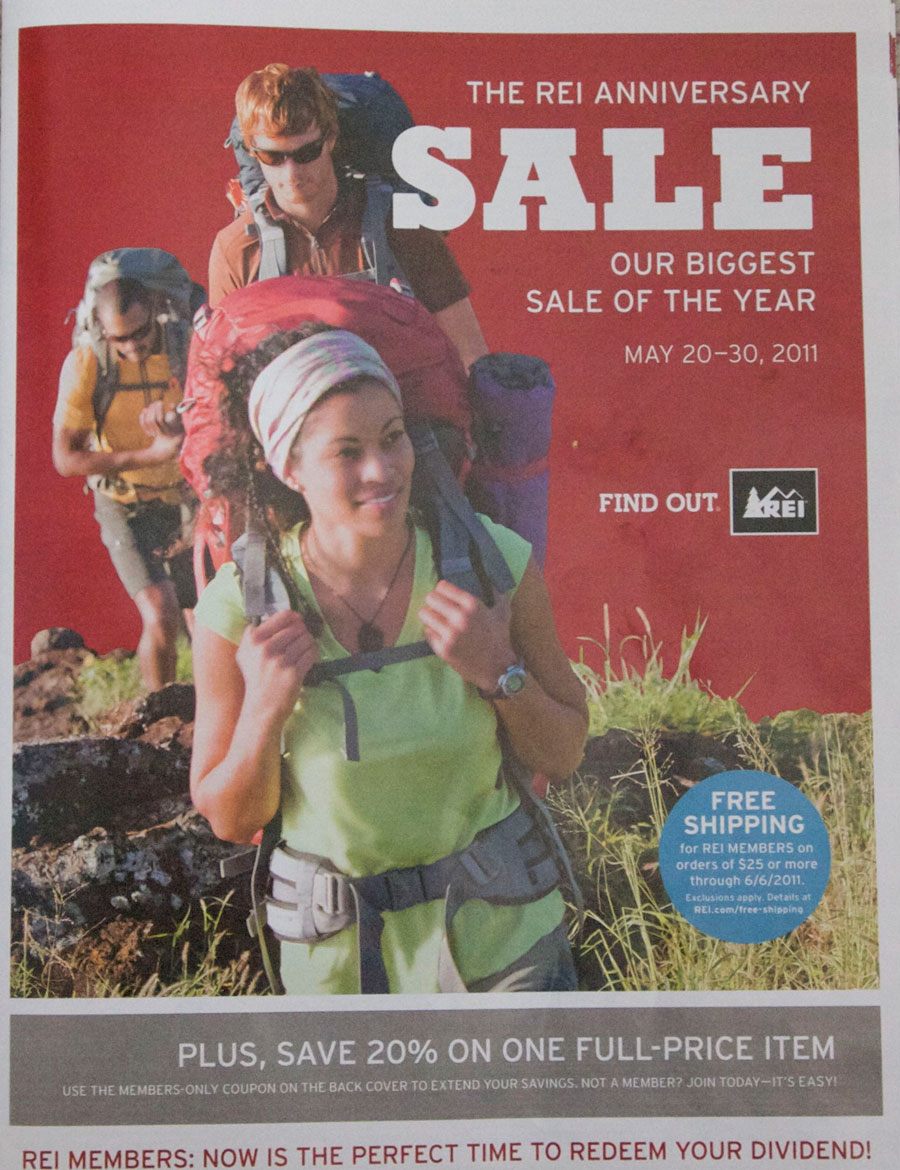This image is an advertisement poster featuring a photograph of three hikers walking on hilly terrain. The woman leading the group is wearing a green shirt, a headband, and carrying a red hiking pack with something purple attached to its right side. Two men follow behind her. All three hikers are smiling. On the right side of the image, there is prominent text that reads, "REI Anniversary Sale," highlighting it as "Our biggest sale of the year," running from May 20 to May 30, 2011. Below this, a blue circle indicates "Free shipping for REI members on orders of $25 or more through 6-6-2011," with exclusions applying and further details available at REI.com/freeshipping. A horizontal gray strip beneath the image states, "Plus save 20% on one full price item," and an announcement in red letters encourages REI members to redeem their dividend: "REI members, now is the perfect time to redeem your dividend." Additional text promotes using a members-only coupon on the back cover to extend savings and invites non-members to join REI.